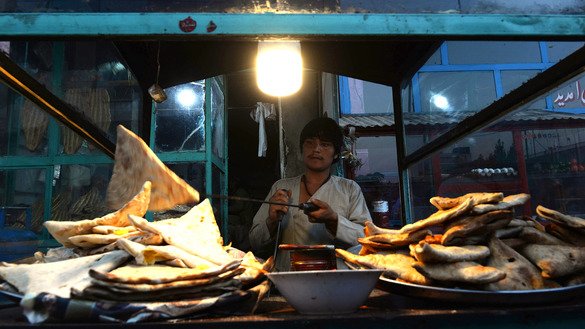The image captures a clear and well-lit scene of an Asian man, likely a street food vendor, dressed in a white v-neck shirt and standing behind a counter. He is holding a silver skewer that has a triangular, dough-like substance on it, possibly flatbread. The counter features two large plates of food, one directly in front of him with more of the dough-like substance, and another plate to the right with a different type of food, possibly fish. A white bowl is placed between the two plates. The vendor appears to be positioned outdoors, with an architectural background featuring buildings, and the setting is framed by an open metal structure. Above him, a bright yellow light bulb illuminates the area, enhancing the clarity and detail of the scene.